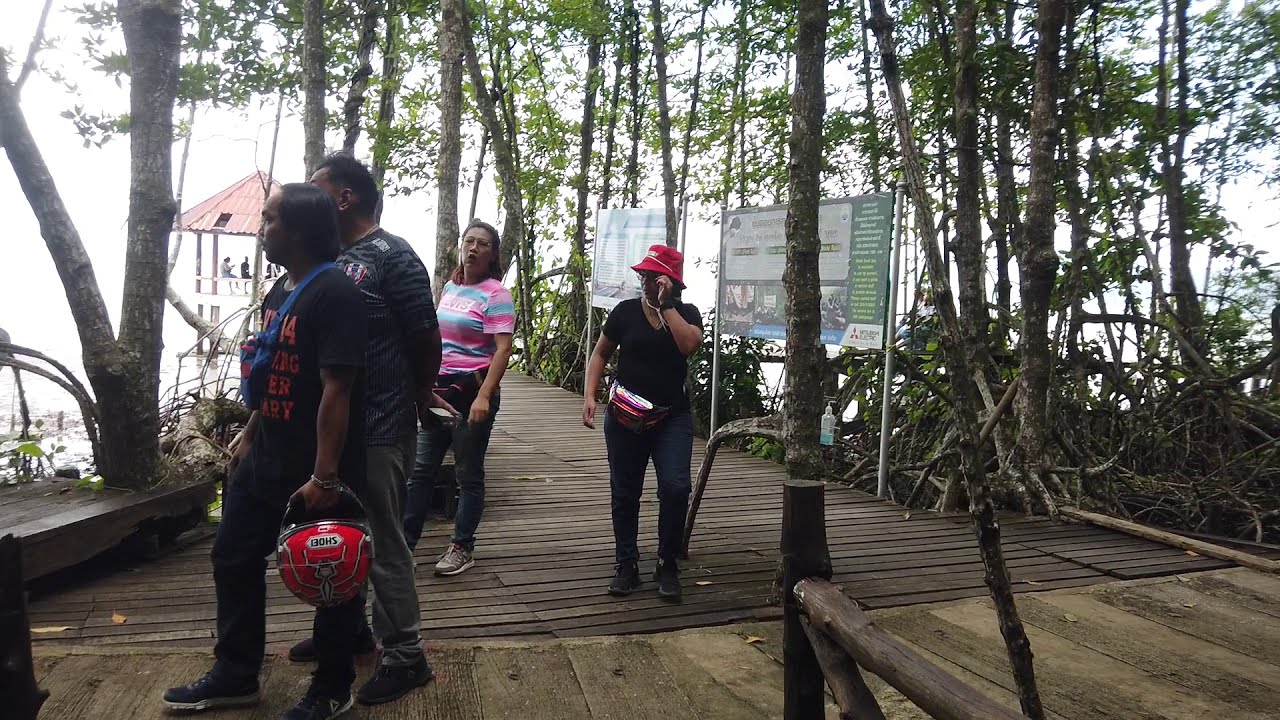The image is a clear outdoor photograph taken in a landscape orientation, depicting a lively scene on a wooden boardwalk surrounded by lush trees. The boardwalk, made of wood planks, extends into the distance where a round pier with a red tile roof can be seen, providing shade for several people sitting underneath. 

In the foreground, four individuals are walking. The person at the front, dressed in cycling attire, holds a red motorcycle helmet in their left hand and has a blue body bag slung across their shoulder. Beside them, a wooden bench is visible on the left side of the image. To the right, a man wearing a red hat appears to be talking on a cell phone, with a pink-striped-shirted woman standing to his left.

Further in the background, an additional two or three people can be seen on the boardwalk. The surroundings are rich with trees, and a hint of water is visible to the left, suggesting a natural, serene setting. There are two signs along the boardwalk, one resembling a billboard, although the text is blurry and unreadable. The bright daylight and the overall clarity of the image highlight this vibrant, possibly touristic scene.

Most of the people appear to be of Asian descent, indicating that this may be a location in Southeast Asia, such as Vietnam or Thailand. The image is characterized by photographic representational realism, capturing a moment of life on this picturesque nature walkway.